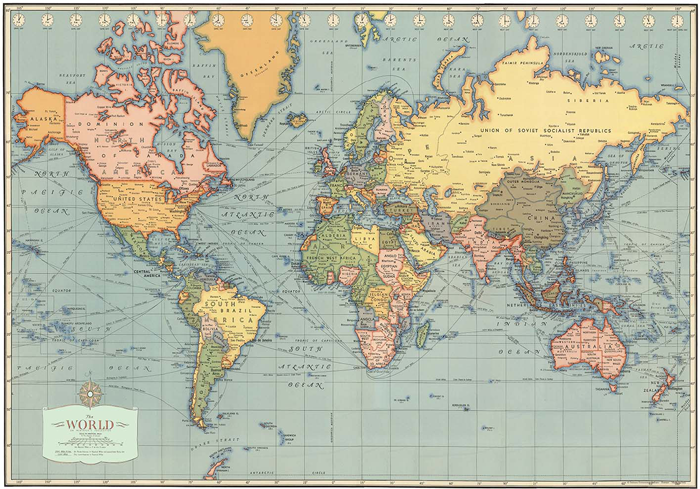This detailed photograph depicts an older, rectangular world map with a bluish-gray sea, presenting a colorful division of continents and countries. Each country is uniquely colored, with the United States in orange, Canada in pink, and Mexico in green. The map is thoroughly labeled, indicating countries, some capital cities, and important rivers. Notably, it lists the USSR under its former name, the Union of Soviet Socialist Republics, suggesting its age. At the top, a row of clocks displays various global time zones, though Hawaii is absent. The map includes grids for latitude and longitude, offering a comprehensive view reminiscent of a classic gaming board.